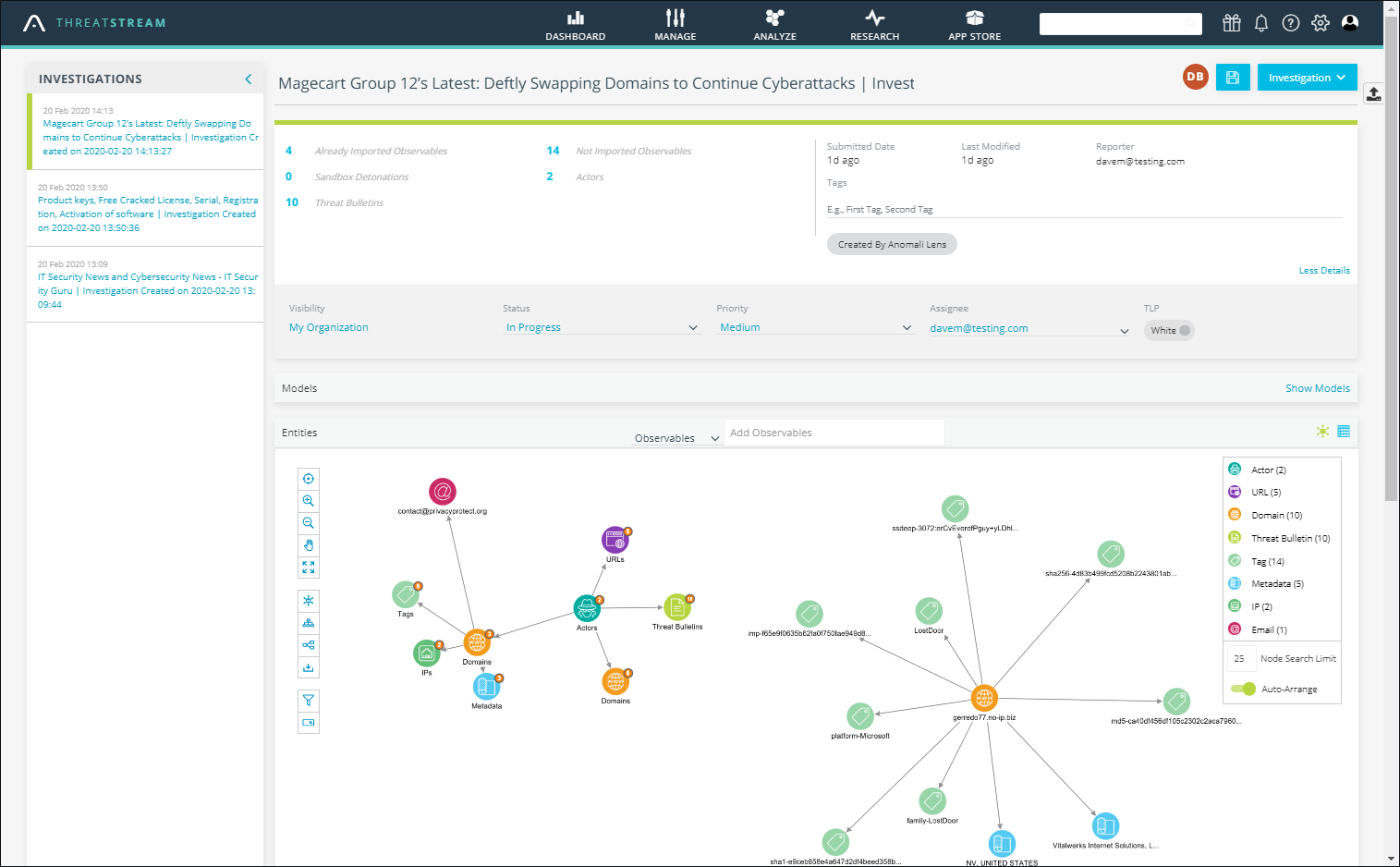The image is a screenshot taken off a computer screen. At the top of the screen, there is a prominent black stripe, with the words "Threat Stream" displayed in the upper right-hand corner. Below this, the interface features a graphical dashboard with tabs labeled "Dashboard," "Manage," "Analyze," "Research," and "App Store." On the left-hand side, the screen shows the section titled "Investigations" prominently at the top.

The center of the screen is dominated by an informational text, labeled "Magecart Group 12's Latest Deftly Swapping Domains to Continue Cyberattacks. Invest." Below this title, the screen features several small, interconnected circles, which are part of two diagrams representing a network. Each circle is connected by lines and is color-coded and labeled with terms such as "URLs," "Actors," "Threat Bulletins," and "Domains." To the right of these diagrams, a small key explains what each type of circle represents. The overall layout suggests a detailed analysis of a cyber threat investigation, showcasing various elements and their interconnections.